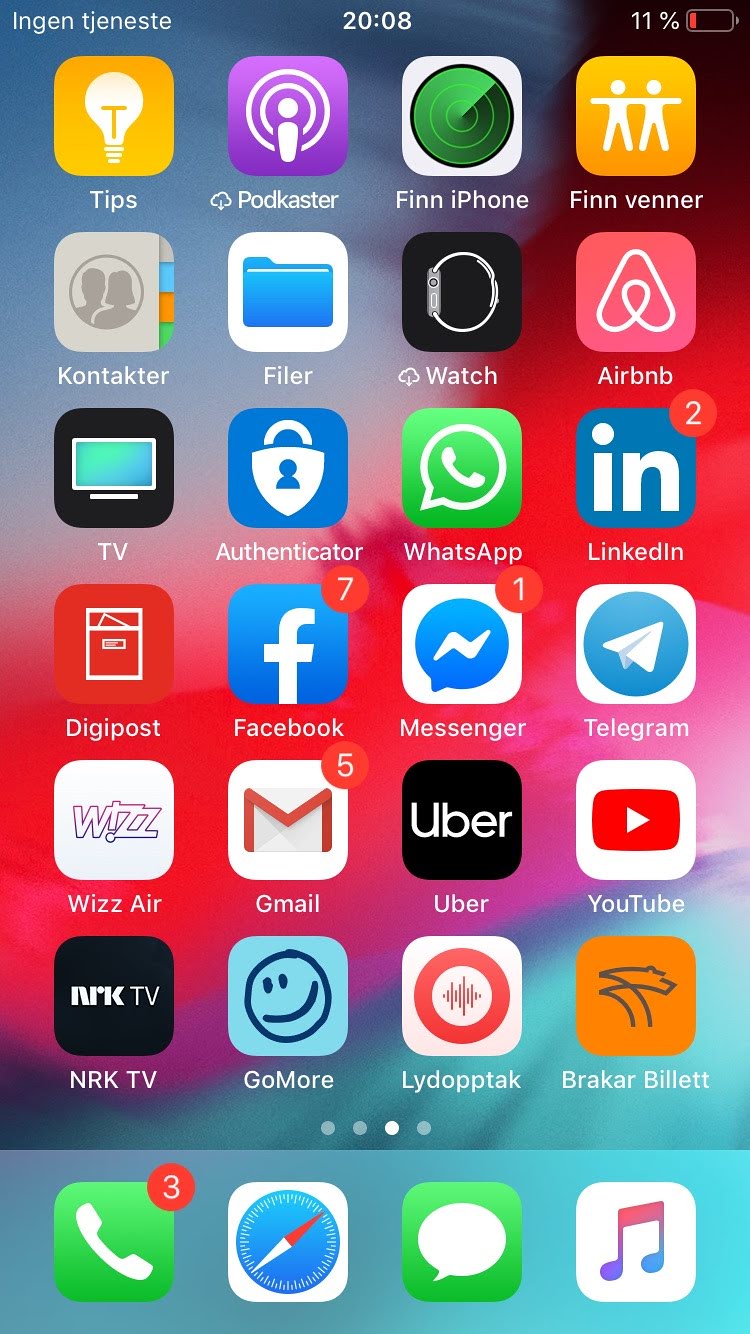The image showcases the home screen of an iPhone. At the top left corner, the network signal icon displays text in a language other than English, appearing as "InGen TNST". The time in the center of the status bar reads 20:08, indicating it is 8:08 PM. On the top right, the battery icon is critically low at 11%, highlighted by a red bar.

The screen contains six rows of app icons, with four apps per row, making a total of 24 apps displayed in rows. At the bottom of the screen, there are four staple iPhone apps situated on the dock. From left to right, these include:

1. The Phone app, characterized by a green square with a white phone icon, and a red notification badge showing 3 missed calls.
2. The Safari app, represented by a blue and white compass icon.
3. The Messages app, a green square featuring a white speech bubble.
4. The Music app, identified by a red background with a white musical note.

Among the apps visible on the main screen are several well-known applications including:
- Find My iPhone
- Airbnb
- LinkedIn
- WhatsApp
- Facebook
- YouTube
- Uber
- Gmail
- Messenger
- Contacts

This detailed display represents a typical, well-organized app layout for a user with diverse utility and social networking needs.